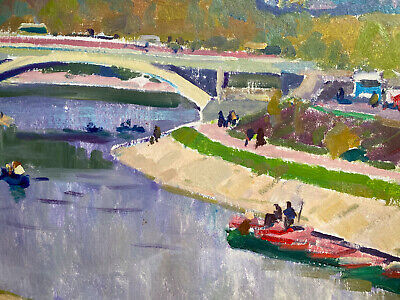This image is a vibrant and colorful painting of a riverside cityscape, depicting a bustling dock area. The painting, potentially created with watercolors, captures the essence of a lively small town with a blend of different hues and shades to create a rich dimension. In the foreground, one can see a blue river with various boats sailing, including a person canoeing and someone on a barge. Alongside the river, a walkway with people strolling reflects a well-landscaped area with trees in green and yellow tones. The scene is accentuated by an arch bridge that spans over the river, adding an architectural element to the mid-ground. Additionally, a painted road with cars runs horizontally across the upper area of the image. In the background, mountains enhance the scenic beauty, creating a sense of depth and tranquility.